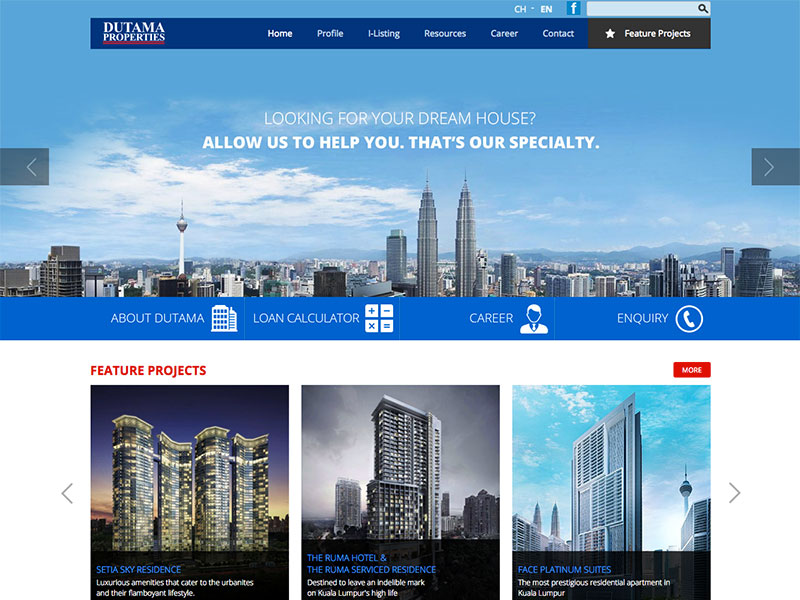The screenshot of the website features a visually striking header with a large cityscape photograph, likely of Seattle, showcasing iconic skyscrapers and the Space Needle against a backdrop of a vibrant blue sky scattered with white clouds. Overlaying the top section of this image is a navigation bar. On the left side of this bar, a blue rectangle displays the text "Dutama Properties" in white font. Spanning the right side of the bar are menu options: "Home," "Profile," "iListing," "Resources," "Career," and "Contact," with "Home" currently selected. To the far right, there is a search field embellished with a black magnifying glass icon.

Directly beneath the search field is a brown rectangle featuring a white five-pointed star and the label "Feature Projects." Centrally aligned across the photo within the sky, a bold white font reads, "Looking for your dream house? Allow us to help you. That's our specialty."

At the very bottom of the photo, a lighter blue rectangle displays additional options in white font: "About Dutama," accompanied by an icon of a skyscraper; "Loan Calculator," with a calculator icon; "Career," alongside an icon of a man; and "Enquiry," paired with a phone icon.